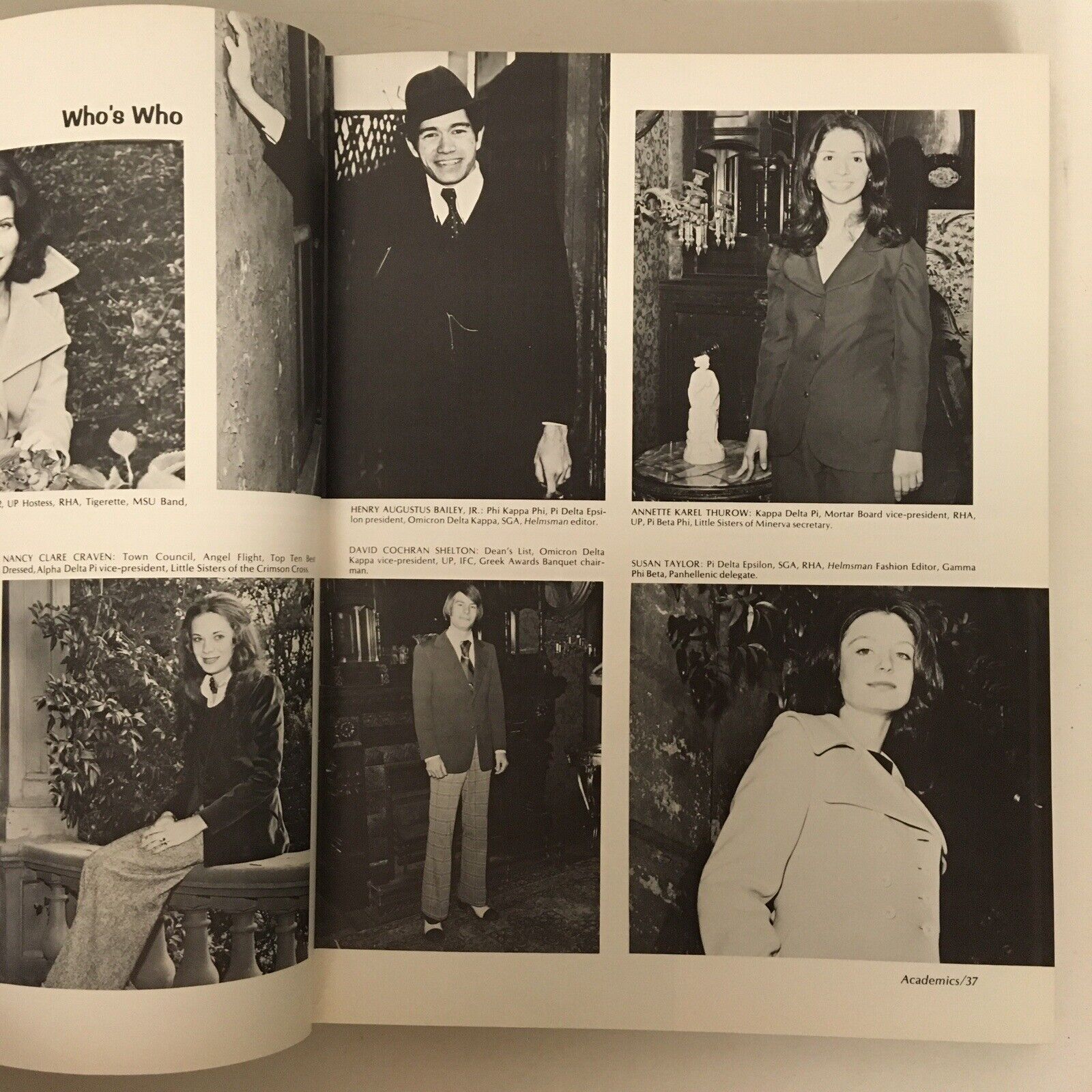This image depicts a black-and-white photograph of an old yearbook, open to pages 36 and 37. The left page is partially visible, revealing the heading "Who's Who?" in the upper left-hand corner. This section appears to feature prominent individuals, possibly members of the school's administration, professors, or notable students, showcasing their involvement in various groups and activities.

On the left page, there are multiple images of well-dressed men and women, detailed in their names and affiliations, such as clubs and academic roles. Notably, three females and two males are fully visible, with one additional female only partially shown as a third of her face is obscured. Their attire, consisting of suits and long coats, and their vintage hairstyles, suggest the yearbook is from an earlier era. The open pages highlight the meticulous presentation of these individuals, each captured in different locations around the campus.

The right page, which we can see entirely, continues this theme with neatly arranged photos—three on the top row and three on the bottom. Captions accompany these photos, though they are not clearly legible. Central to the layout is a man in a dark suit and hat, smiling with one hand propped against a wall. Next to him stands a woman in a suit, positioned beside a round table with a small statue, also smiling. Below them are three more individuals—two women and one man—each dressed in formal attire, offering a glimpse into the distinguished presentation of the yearbook's subject matter. The page number "37" marks the end page visible.